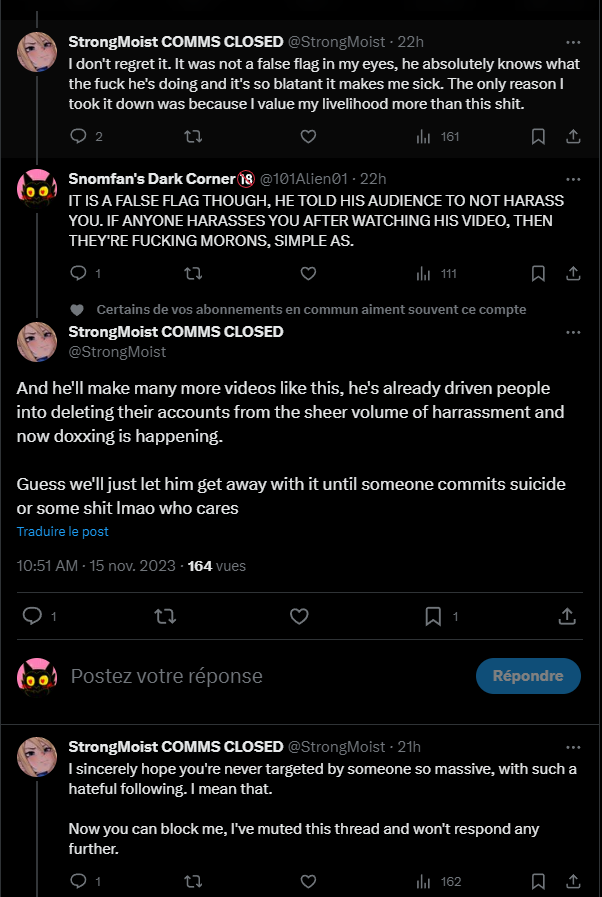A detailed screen capture of an ongoing chat conversation between two users, @strongmoist and @snowmfansdarkcorner (referencing @101alien01), reveals heated exchanges about online harassment. @strongmoist expresses frustration, asserting, "I don't regret it. It was not a false flag in my eyes. He absolutely knows what he's doing, and it's so blatant it makes me sick. The only reason I took it down was because I value my livelihood more than this." In response, @snowmfansdarkcorner contends, "It is a false flag though. He told his audience not to harass you. If anyone harasses you after watching his video, then they're morons, simple as." @strongmoist retorts, highlighting the gravity of the situation, "And he'll make many more videos like this. He's already driven people into deleting their accounts from the sheer volume of harassment, and now doxing is happening. Guess we'll just let him get away with it until someone commits suicide or something. LMAO, who cares?"